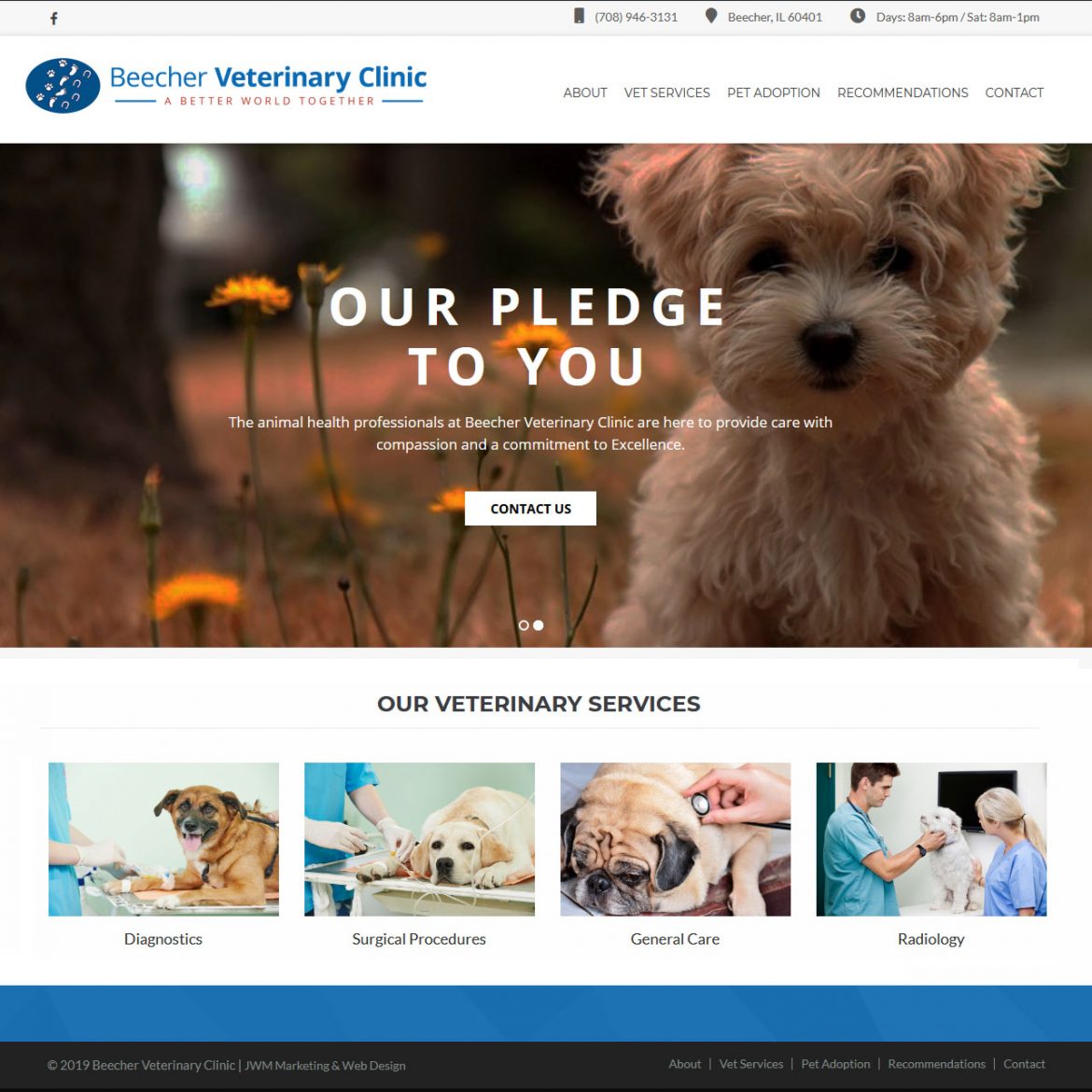The image showcases a header with the contact information "708-946-3131, Beecher, IL 60401," and operating hours "Monday to Friday, 8am-6pm; Saturday, 8am-1pm." A prominent blue oval icon reads "Beecher Veterinary Clinic - Better World Together." Below the header is a menu featuring options for "Vet Services," "Pet Adoption," "Recommendations," and "Contact."

Central to the image is a heartwarming photograph of a white, curly-haired puppy playing in a yard dotted with dandelions. Beneath the image, a pledge from Beecher Veterinary Clinic declares their commitment to providing compassionate and excellent care, emphasizing their dedication as animal health professionals.

A prominent white button labeled "Contact Us" encourages engagement, with additional text detailing their veterinary services, including "Diagnostics," "Surgical Procedures," "General Care," and "Radiology."